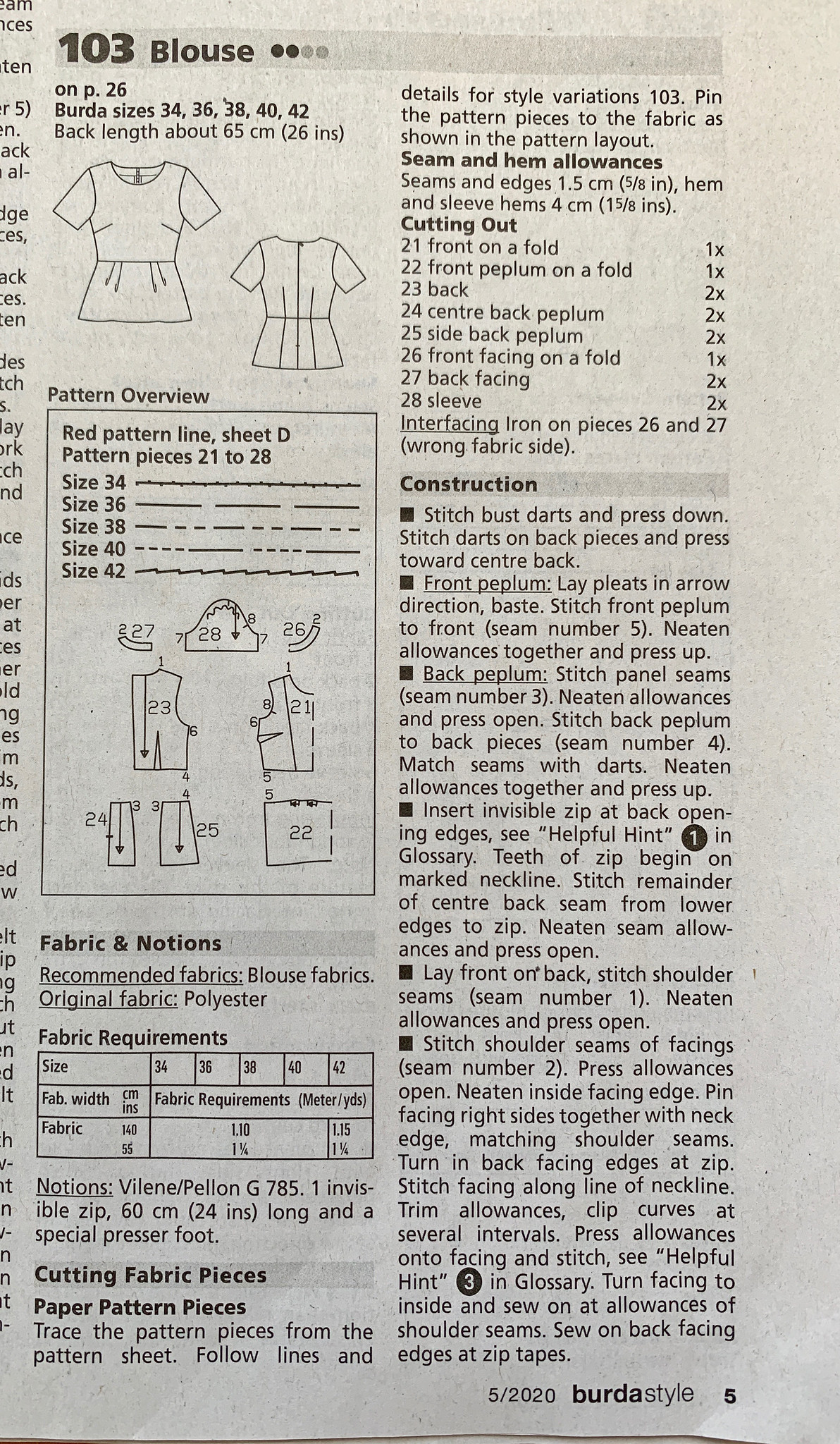This image depicts a page from the May 2020 issue of "Burda Style" magazine, specifically page 26. The page is dedicated to Pattern 103, a blouse available in sizes 34, 36, 38, 40, and 42, with a back length of approximately 65 centimeters (26 inches). The background is white with black printed text and features two sections. 

On the top left, there are simplistic black outline drawings showing the front and back views of the blouse, which has a bottom curve similar to a miniskirt. Below these illustrations, a rectangular section provides a pattern overview, detailing "Red Pattern Line Sheet D" with pattern pieces numbered 21 to 28. 

The page is divided into categories such as "Fabric and Notions," "Recommended Fabrics," "Cutting Fabric Pieces," "Paper Pattern Pieces," and "Cutting Out and Construction." Each category includes bold headings and detailed instructions for sewing the blouse. The right side of the page continues with headings like "Seam and Hem Allowances," and "Construction," offering elaborate steps for assembly. In the bottom right corner, the number 5 and the text "Burda Style" are present, indicating the specific edition details.